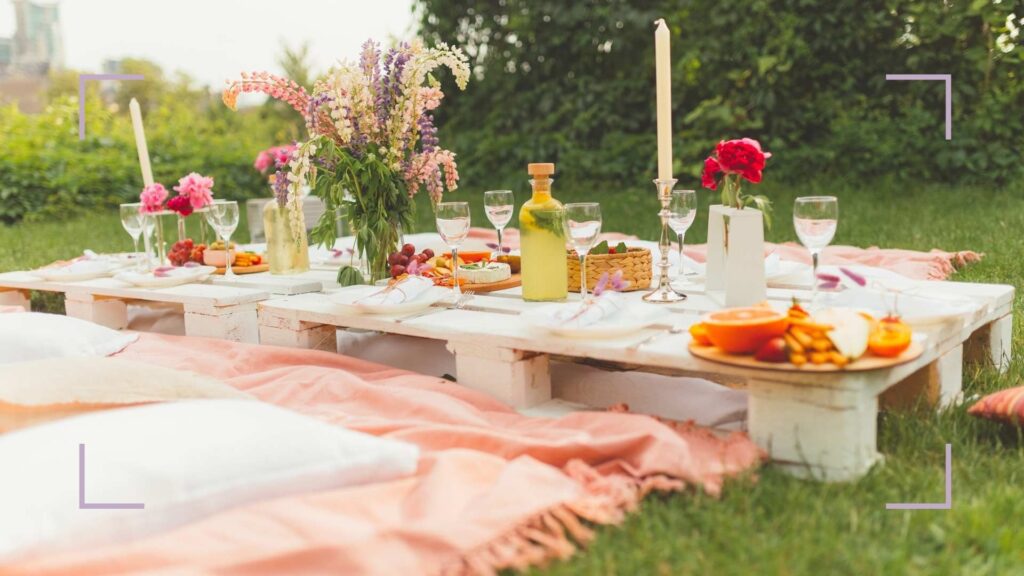This photograph captures a luxurious midday picnic set in an open field surrounded by lush greenery. The focal point is an elegantly arranged, low table crafted from white-painted wooden shipping pallets. The table is adorned with various glassware, including wine glasses filled with clear liquid and a glass bottle of lemonade. Set amidst the arrangement are lit candles, adding a warm, inviting ambiance.

In the center of the table, a tall vase holds a vibrant bouquet of pink and purple flowers. The table is also decorated with plates that have cloth napkins, cut fruit, and baskets of assorted snacks such as fruits, crackers, and cheese. On either side of the table, there are colorful blankets and white pillows, creating a cozy seating area.

The photo is taken during daylight, enhancing the vividness of the greens in the distant trees and the overall lively atmosphere. Subtle details, such as the corner markings akin to a camera viewfinder, frame the image and indicate its deliberate composition. In the distant background, the outlines of buildings can be discerned, suggesting a park-like setting, possibly within an urban or campus environment.